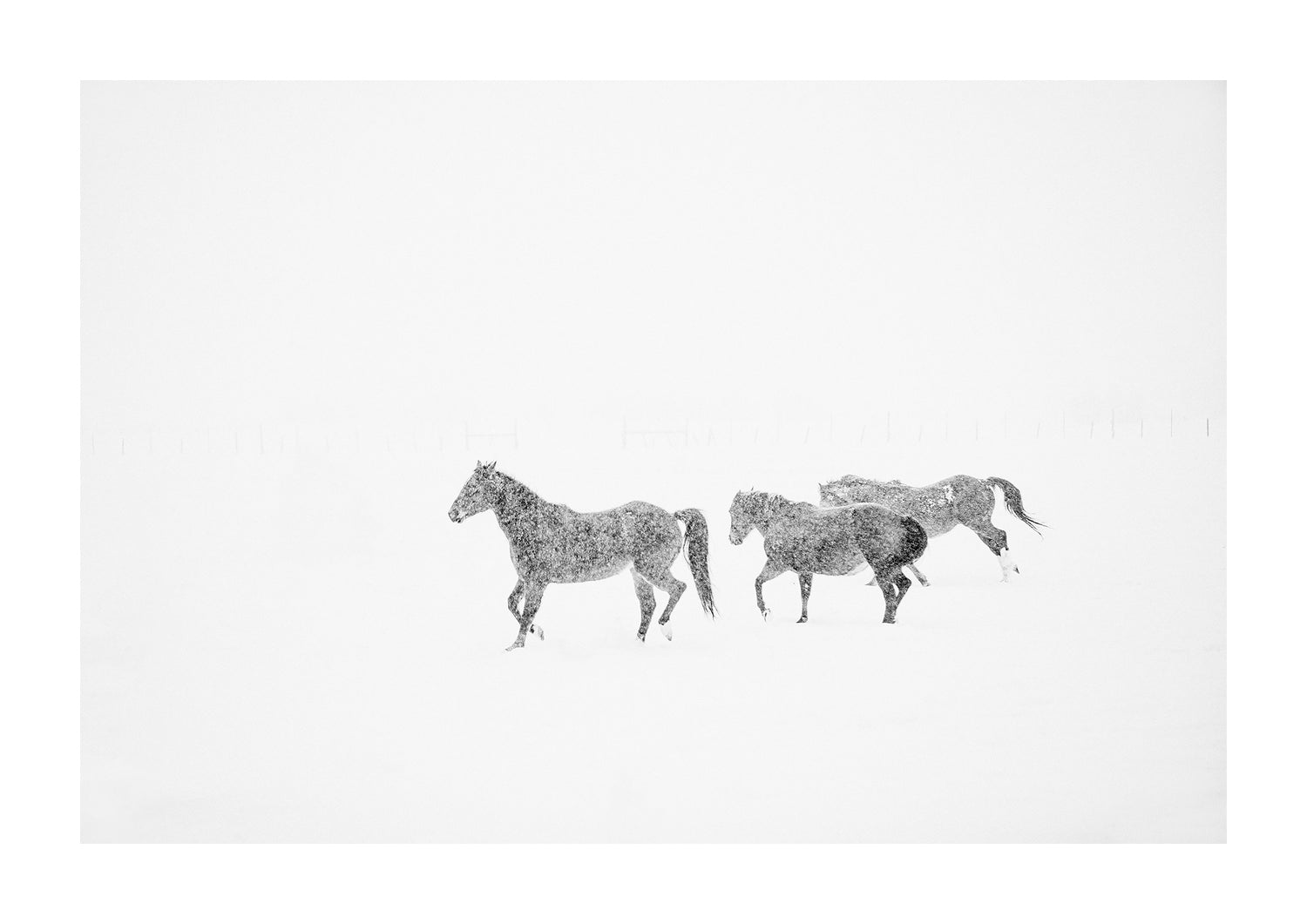In this photograph, we see three black horses amidst a heavy snowfall in a winter scene. The background of the image is an almost pure white, slightly vignetted at the corners, suggesting it was taken during a blizzard. The foreground is scarcely visible, with only the faintest traces of trees discernible. In the center of the image, the trio of horses is captured in motion, appearing as if they are charging forward. The horse in the center has its head raised, while the two behind have their heads lowered. A thick cloud of snow flows in front of them, enveloping their bodies and creating a dramatic, almost ghostly effect. The heavy snowfall between the camera and the horses gives them a fuzzy appearance, akin to television interference. The entire scene is completely washed out, emphasizing the intensity of the blizzard and the ethereal beauty of the moment.